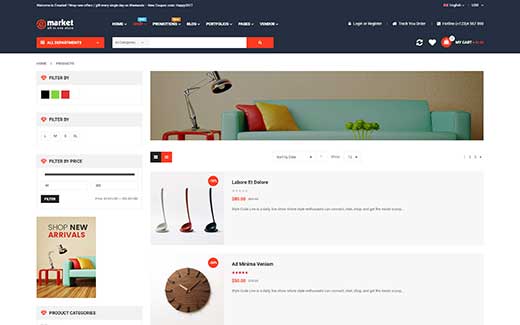The homepage of the Market website features a sleek, modern design with a black banner at the top. In the upper left corner is the website's name, "Market," accompanied by a small red logo. To the right of the logo, there are very small, clickable category labels with drop-down boxes. Below the banner, you will find a search bar with a red arrow button to initiate the search. Adjacent to the search bar, several icons are aligned: a heart, an alert bell, and a refresh button.

The main body of the webpage is presented on a white background. At the top, a large, rectangular image showcases a contemporary blue couch adorned with orange and yellow pillows. To the left of the couch is a silver desk lamp. Below this header image, the webpage displays two products. The product thumbnails are positioned on the left side, with their descriptions enclosed in light gray text boxes to the right. Although the text is too small to read clearly, the first product's image appears to be colorful ladles, while the second product resembles a wooden clock.

Additionally, on the right side of the page, there is a small thumbnail of a poster that promotes "Shop New Arrivals." This poster features the same image of the blue couch with orange and yellow pillows, giving a consistent visual theme to the homepage.